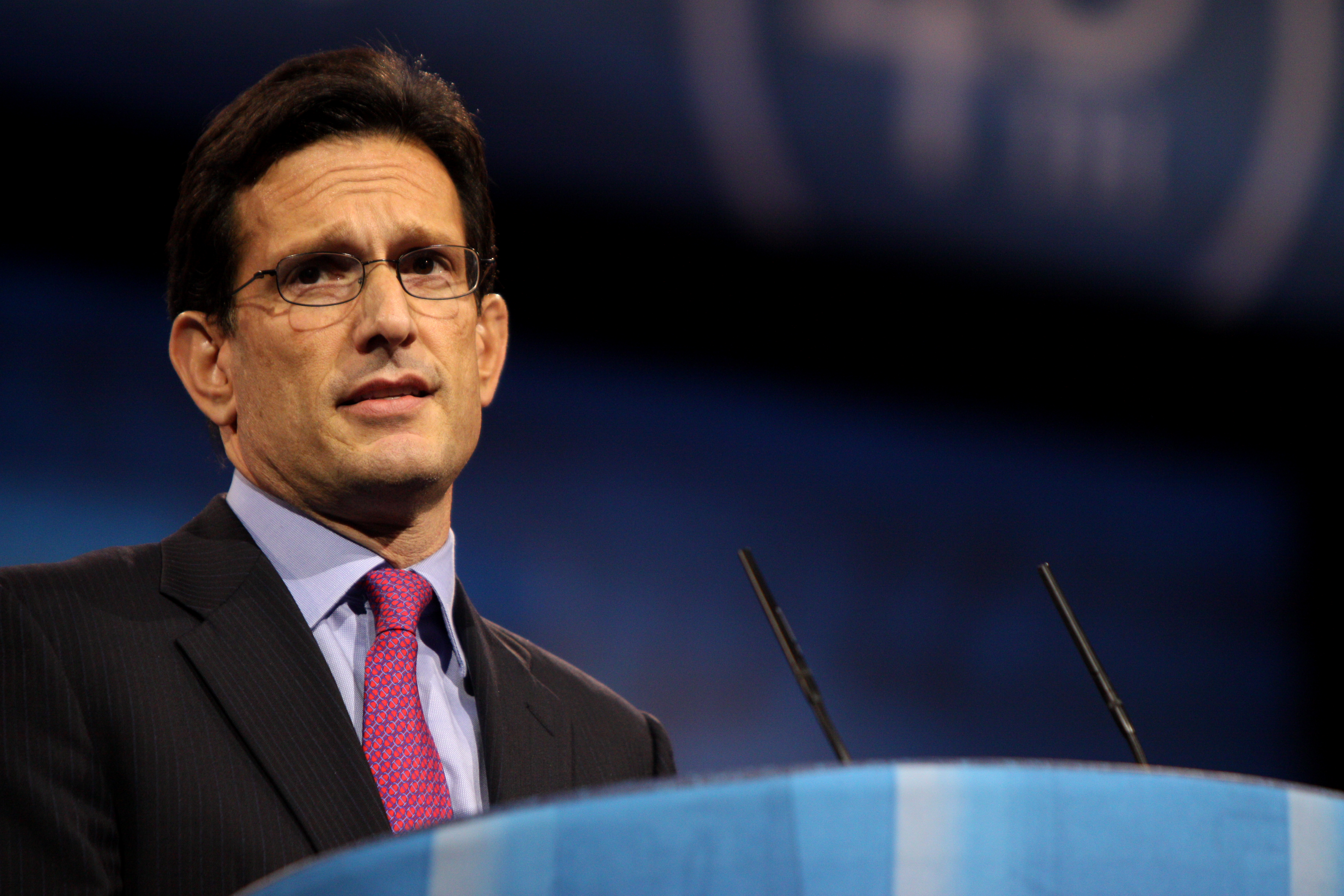In this indoor image, the background is generally out of focus, preventing us from discerning specific details, although it does appear to be an indoor setting. Centered towards the left of the frame, a podium is visible at the bottom of the image, equipped with a microphone. In front of the podium stands a middle-aged man dressed in a sleek suit, seemingly in the midst of delivering a speech. The atmosphere is formal, with no text visible anywhere in the image. The colors present in the scene range from various shades of light blue, white, gray, off-white, black, red, tan, and dark blue. The overall composition and elements suggest an event or conference setting.